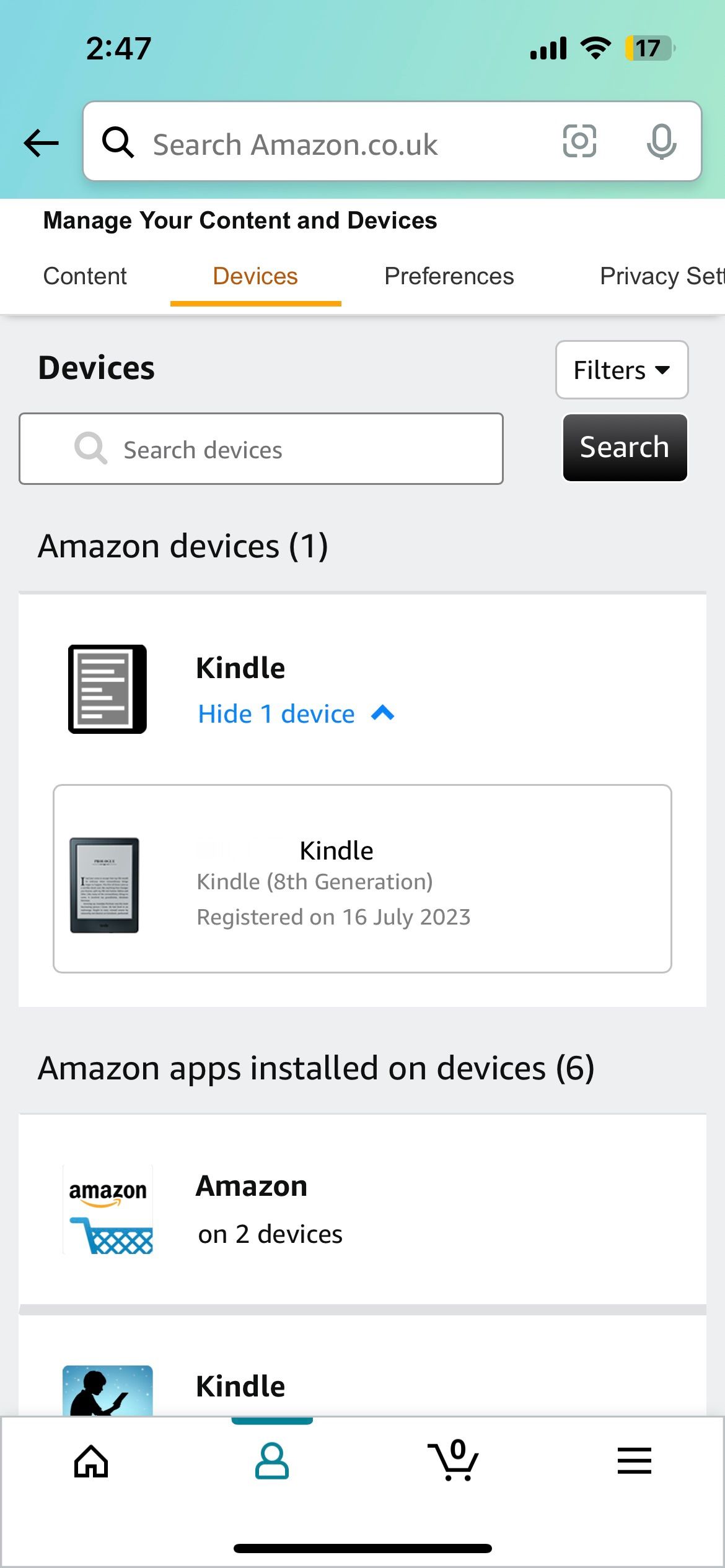The image is a screenshot taken on a smartphone displaying the "Manage Your Content and Devices" section of the Amazon.co.uk website. Various elements located in the typical smartphone interface, such as the time, network strength, and battery level icons, are visible along the top of the screen. Below them, the Amazon URL is prominently displayed along with a search bar.

The main section of the screenshot features the yellow-highlighted "Devices" tab under the "Manage Your Content and Devices" header. The section reveals that the user owns one Amazon device, a Kindle, as indicated by the title "Devices."

Further down the page, the "Amazon apps installed on devices" section shows six apps in total, although only the first two are visible within this screenshot. The visible apps include the Amazon main shopping app and the Kindle app, both represented by their respective icons located to the left.

Towards the bottom of the screen, three navigational icons are also visible: the "Home" icon on the left, the "Person" icon in the middle (which is highlighted), and the "Cart" icon on the right. Additionally, a menu icon with three horizontal lines indicating more settings and navigation options is also visible within this section of the interface.